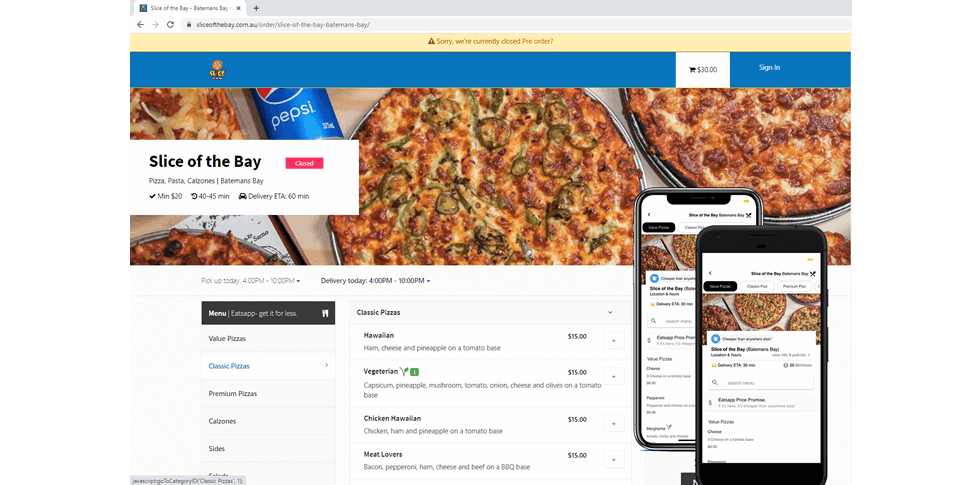This screenshot captures a pizza delivery website. At the top, a browser tab is open, titled "Slice of the Day," with the corresponding URL beneath it. A large yellow banner prominently states, "Sorry, we are currently closed. Pre-order?" with an interactive link. Above this, a blue banner displays a notice: "$30" with a "Sign In" button.

The central section features a large promotional image showcasing four different pizzas and a can of Pepsi. Overlaid text reads, "Slice of the Day closed in Pizza Pots Calzones Bateman’s Bay, minimum $20, 40 to 45 minutes delivery, ETA 60 minutes."

Adjacent to the main imagery, there are smaller images of mobile phones, each mirroring the ordering information displayed on the desktop site. 

Below these images, the menu options are detailed: Value Pizzas, Classic Pizzas, Premium Pizzas, Calzones, and Sides. The "Classic Pizzas" category is currently selected, listing options such as Hawaiian, Vegetarian, Chicken Hawaiian, and Meat Lovers, each priced at $15.

Although it's difficult to discern which items have been added to the cart, a $30 total indicates some selections have already been made.